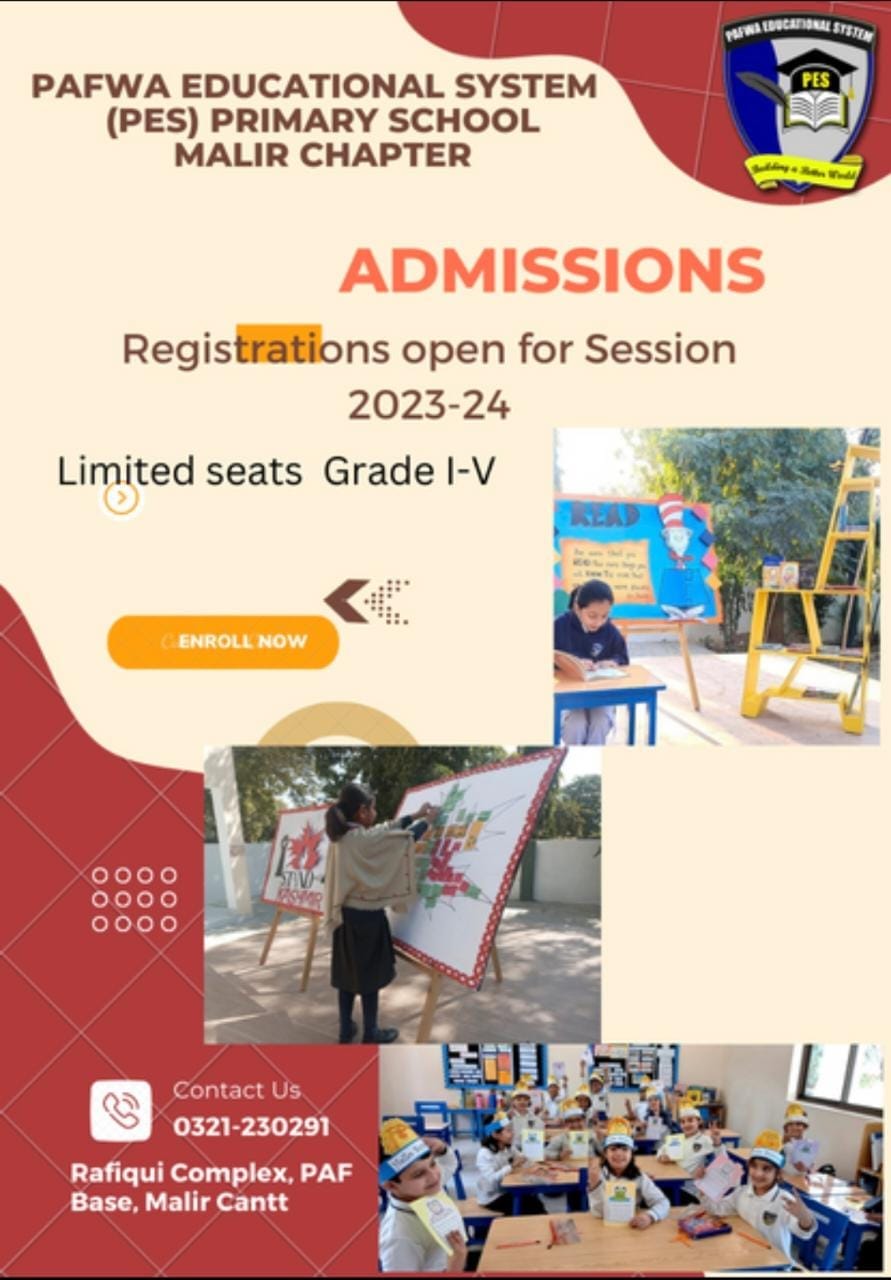The image is an advertisement for the PAFWA Educational System, specifically for PES Primary School, Malheur Chapter. The top of the image prominently features the school’s name. On the right side, there's a corner colored red, displaying a blue and gray shield with a yellow banner at the bottom and a feather sticking out of a book, with the initials “PBS” above it. 

Centered in bold capital letters is the word "ADMISSIONS," indicating the purpose of the advertisement. Below this, the text announces, "Registration Open for Season 2023 to 2024, Limited Seats, Grade I-V," emphasizing the urgency and exclusivity of the enrollment opportunity. Arrows pointing left underline the phrase "Enroll Now," encouraging immediate action. Following this call to action is the directive to "Contact Us" for further information.

Beneath these textual elements, there are three small pictures of students engaged in various school activities, showcasing the dynamic and educational environment of the school.